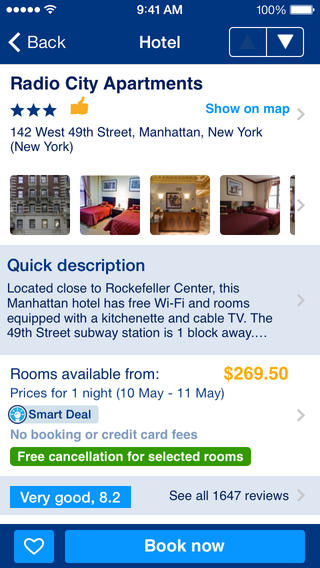This image is a screenshot of a mobile device displaying hotel information. In the top left corner of the screen, there are indicators for network connectivity, showing the signal strength at 5 out of 5 bars and Wi-Fi strength at 3 out of 3 bars. Centered at the top of the screen, the current time is displayed as 9:41 AM. On the top right, the battery level is shown to be fully charged at 100%.

In the main content area, there is text providing details about a hotel named "Radio City Apartments," rated with three stars. The text includes an option to "Show on Map" and lists the hotel's address as 142 West 49th Street, Manhattan, New York.

A brief description follows, stating: "Located close to Rockefeller Center, this Manhattan hotel offers free Wi-Fi and rooms equipped with a kitchenette and cable TV. The 49th Street subway station is one block away."